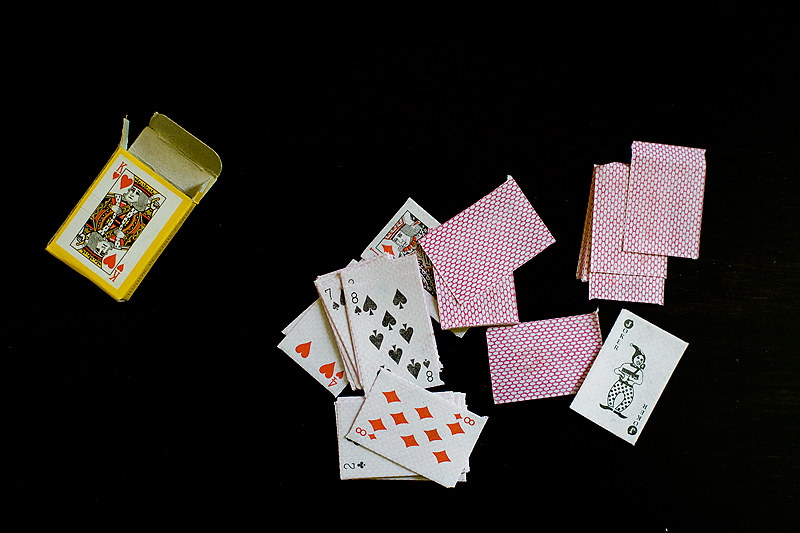In the center of the image, a scattered deck of playing cards is artfully strewn across a black background, creating a striking contrast. The scene is punctuated by a yellow-bordered card box, positioned diagonally with its bottom left corner entering from the left side of the frame about midway from top to bottom, and its bottom right corner extending downward to the right. The card box is open, revealing its light brown interior folds with two flaps standing upright. Peeking out of the box is the Red King card, adding a pop of color to the composition.

Directly below the open box, the cards begin their scattered arrangement. The first visible card is the Four of Hearts, angled downward to the left and partially covered by a small stack of approximately 20 cards. Among this stack, only the Seven of Spades and the Eight of Spades are fully discernible. Beneath these cards and slightly to the right lies the Jack of Diamonds, topped by two other cards – one positioned vertically at the bottom and the other diagonally crossing from the right down to the left.

Further down to the right, one card reveals its back, which is red and white in color, matching the reverse design seen throughout the image. Just below this is another card stack, prominently showing the Two of Clubs turned horizontally, with the Eight of Diamonds placed diagonally atop it. To the right of the card with the visible back, a black Joker card is angled up and to the right, just overlapping the corner.

Above the Joker, another small pile of cards is visible from the reverse side, one of which is slightly pulled out toward the bottom. Adjacent to this pile and slightly overlapping to the right, another collection of cards creates a layered and dynamic composition.